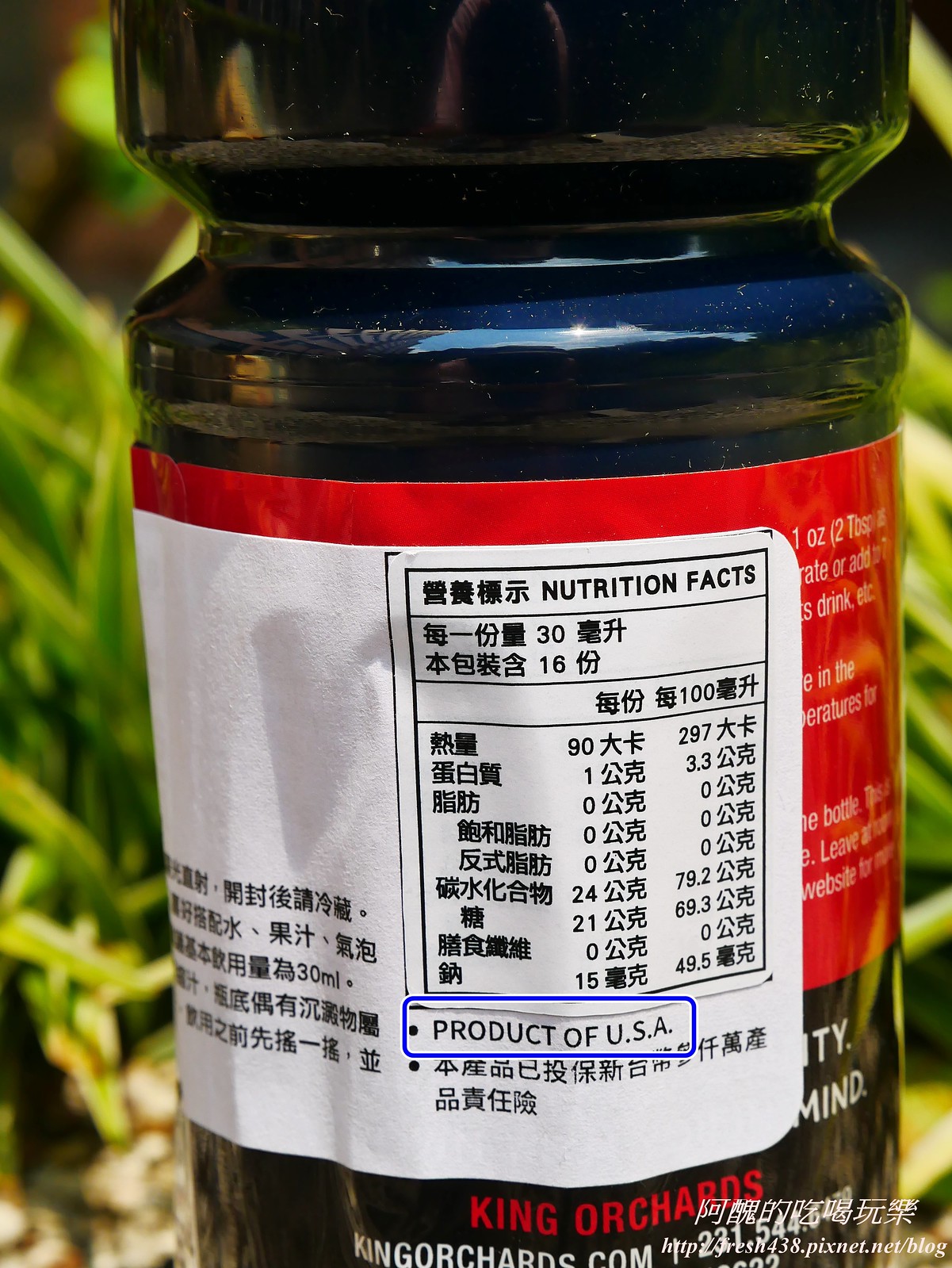This image displays a glass jar, predominantly black with a cylindrical shape that curves inward slightly at the top before flaring out again. The jar features two prominent labels: a primary red label reading "King Orchards" and "kingorchards.com" partially obscured by a white label overlay. The white label wraps around the side and back and is primarily covered in Asian characters, with the only English text being "Nutrition Facts" and "Product of USA." The "Product of USA" text is distinctly highlighted by a blue outlined rectangle likely added by the person viewing the image. The backdrop reveals some grass or reeds, adding to the natural ambiance of the scene.